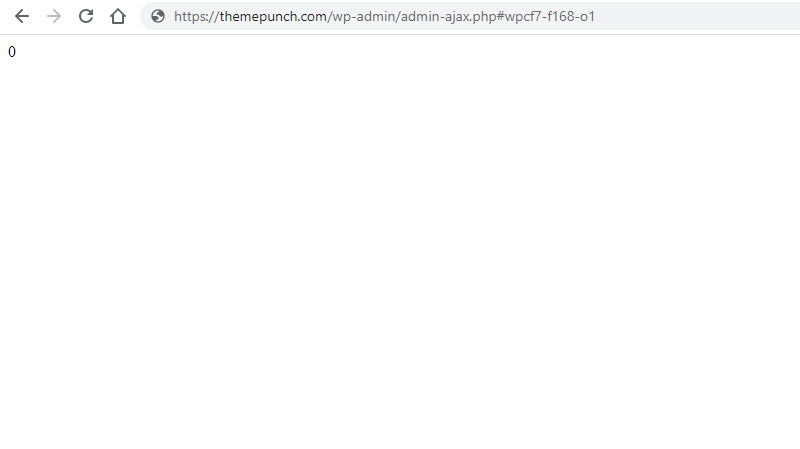In this screenshot, we see a minimalist image primarily featuring a white screen. The main focus of the image is the browser's header, which includes an address bar that is light gray with black text. Inside the address bar, there is a small icon resembling a planet Earth with dark shading, indicating that the page is secure. The URL displayed in the address bar is "https://themepunch.com/wpadmin/admin-ajax.php#wpcf7f16801." At the top left corner of the header, we see a series of navigation icons: a left arrow for moving backward, a right arrow for moving forward, an undo icon, and a home icon. The overall appearance of the image is clean and simple, with the navigation and address bar being the only elements present.